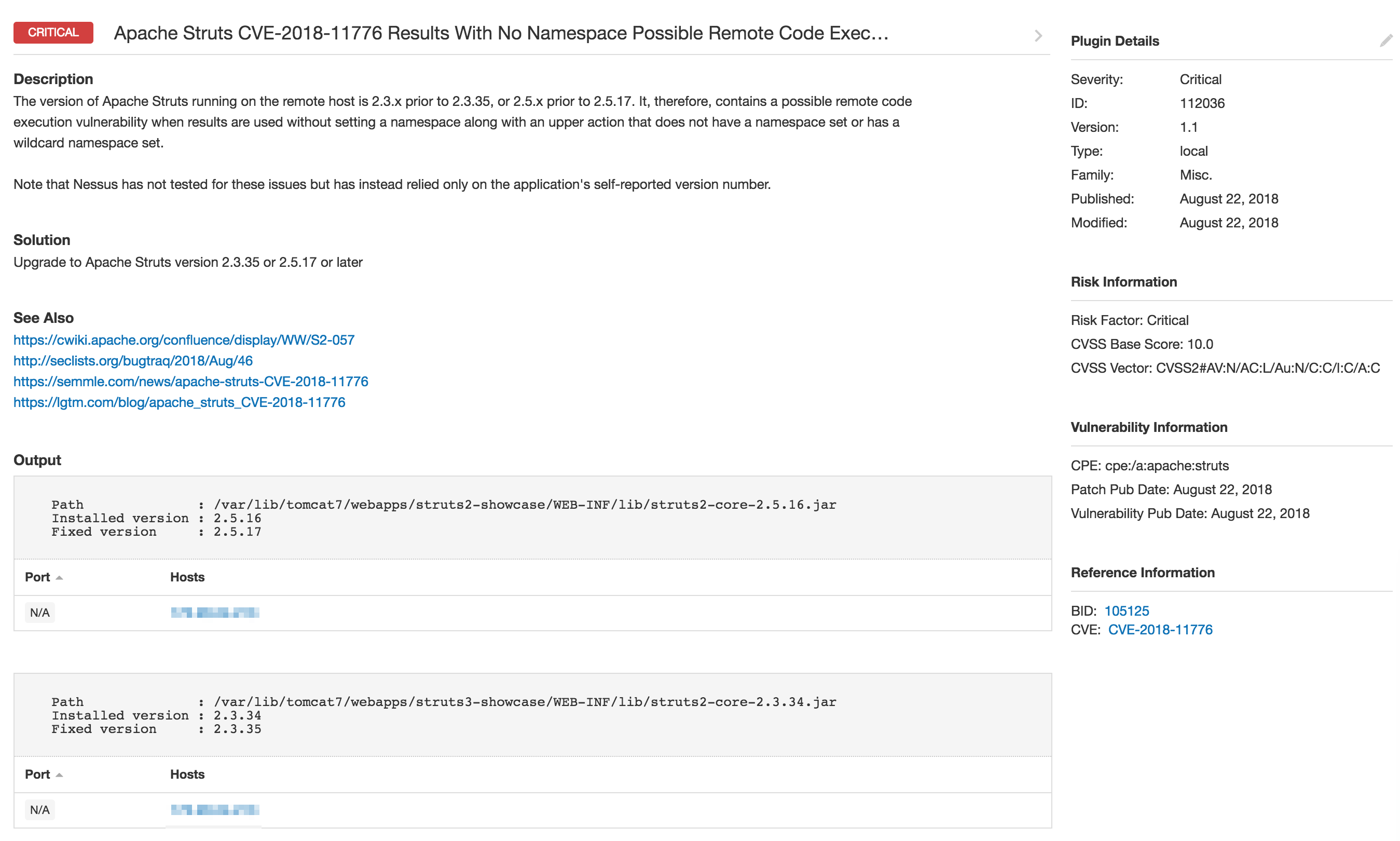**Detailed Caption:**

The screenshot displays a warning page about a critical security vulnerability in an Apache Struts plugin. In the top left corner, a red box highlights the warning title: "Critical Apache Struts CVE-2018-11776." The vulnerability pertains to versions of Apache Struts running on the remote host—specifically, versions 2.3.x prior to 2.3.35 and 2.5.x prior to 2.5.17. 

The warning explains that these versions contain a remote code execution vulnerability when results are used without setting a namespace, in combination with an upper action lacking a namespace or using a wildcard namespace. The advised solution is to upgrade to a newer, patched version of Apache Struts.

For further information, the page provides four additional resource links. An output box beneath the description contains more detailed data about the vulnerability.

On the right side, a column labeled "Severity" categorizes the risk as "Critical." Other details in this column include the vulnerability's ID number, version number, type, family, and both the published and modified dates, which are recorded as August 22, 2018. The risk factor is deemed critical with a CVSS base score of 10.0. The page also includes sections for vulnerability and reference information.